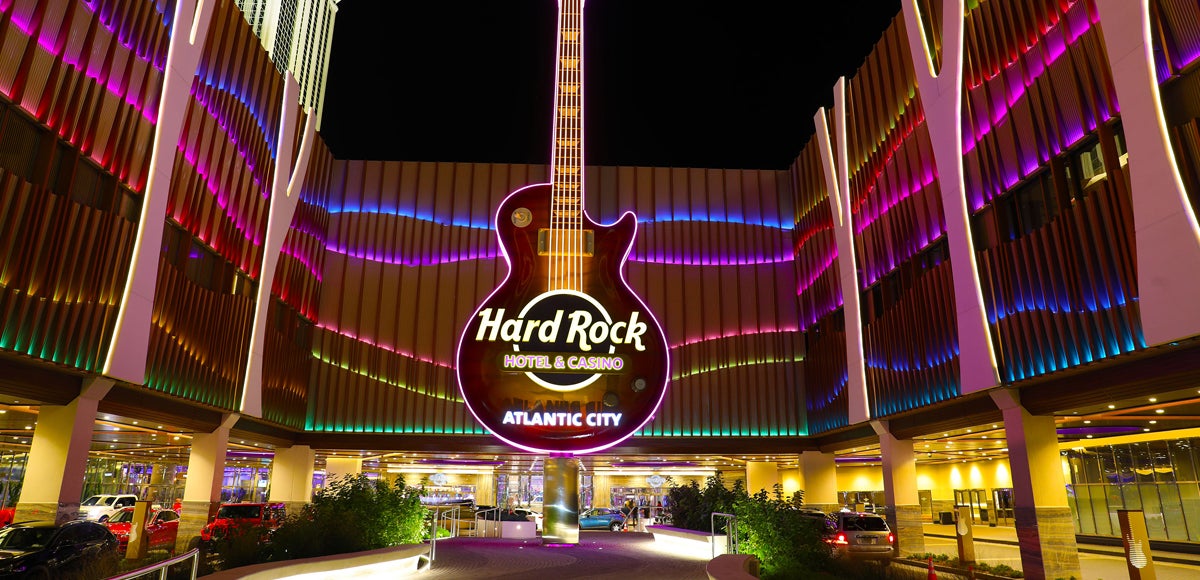This is a vividly detailed nighttime photograph of the Hard Rock Hotel and Casino in Atlantic City. The focal point of the image is a large, electrifying neon-lit guitar that towers above the main entrance, its strings extending dramatically past the roof. The body of the guitar displays the "Hard Rock Hotel and Casino, Atlantic City" logo in striking white lettering. The entire façade is illuminated in a mesmerizing array of neon colors, including hot pink, hot purple, neon green, neon yellow, and neon blue, casting a vibrant glow over the scene. Directly beneath the glitzy entranceway, the glass doors lead into the hotel and casino, flanked by a parking garage on the lower level. Several cars, including a noticeable blue car at the front and red cars to the left, are seen either parked or in the process of dropping off and picking up guests, enhancing the lively ambiance of the place.